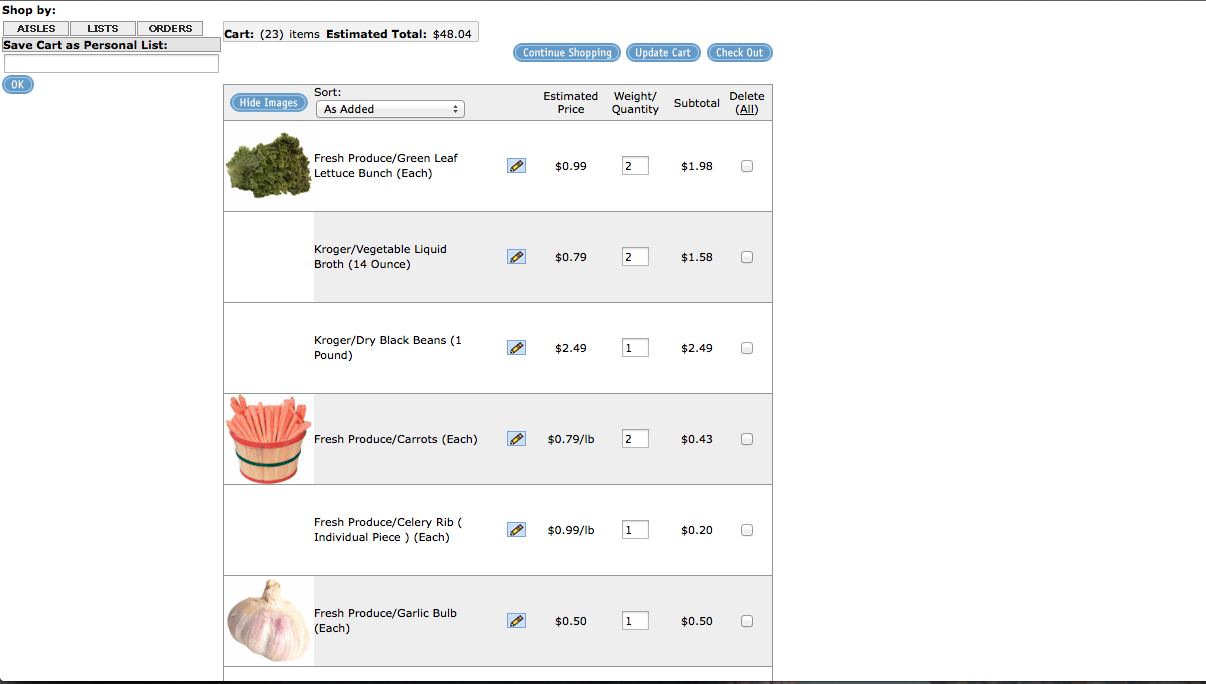In the image, there is an interface resembling a digital grocery shopping list. The top left corner displays options labeled "Shop by" with three buttons underneath: "Aisles," "Lists," and "Orders." Below this is the "Save Card as Personal List" section, where you can type a name and hit "Okay." Currently, there are 23 items in the cart, with an estimated total of $48.04.

The list begins with fresh produce items, starting with lettuce. The estimated price per unit is $0.99, with a selected weight quantity of 2, making the subtotal $1.98. Next to the lettuce entry is a check mark option for deletion, and there is a button at the bottom of the interface allowing for the deletion of all selected items.

Following lettuce, the list includes an entry for Kroger vegetable liquid broth, which is a 14-ounce bottle priced at $0.79 each. With a selected quantity of 2, the subtotal for the broth is $1.58. 

Next is an item for dry black beans, priced at $2.49, with a quantity of 1 chosen. Then, there is an entry showing a barrel of carrots, priced at $0.79 per pound. Two pounds have been selected, resulting in a subtotal of $1.58.

Fresh produce celery ribs are listed for $0.99 per pound, with an entry showing a selection resulting in $0.20 worth. Lastly, for fresh produce, garlic white bulbs are priced at $0.50 each, with one bulb selected.

Overall, the interface features a detailed breakdown of items, with images available for some. The subtotal and weight quantity for each item are clearly listed alongside options to modify or delete items from the cart.